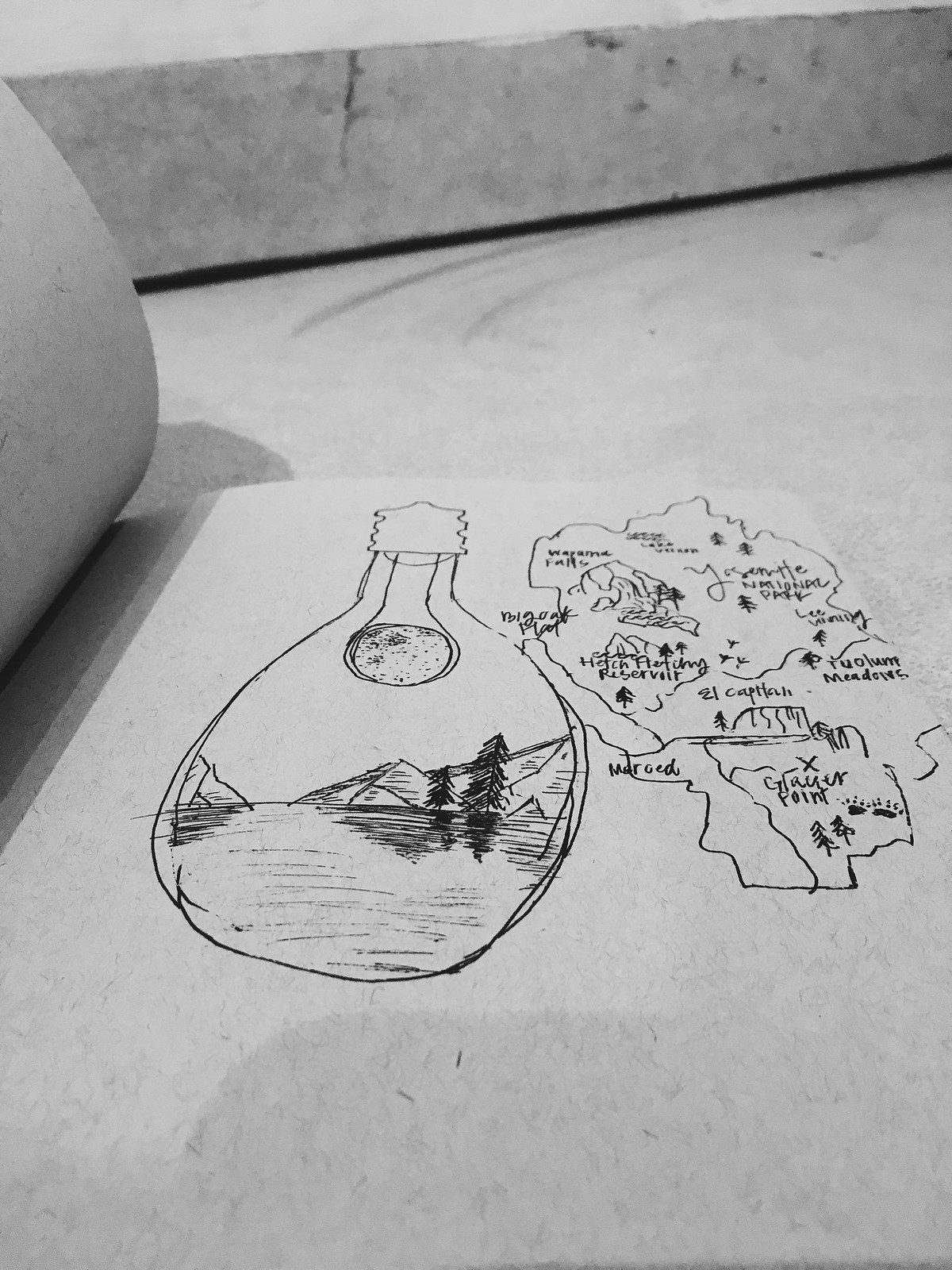The photograph captures a hand-drawn illustration on off-white, fibrous paper within a notebook. The notebook rests on a stone or marble-like surface, which almost matches the paper's color tone, initially creating the illusion that the drawing is directly on the surface. The shadow of the notebook's pages, cast midway up on the left side, reveals its presence, with the curved pages peeking out from the left edge.

The illustration features a conical science beaker with a little, intricately detailed waterfront scene inside, including a lake, mountains, and trees, all rendered in dark pencil shading. Above the beaker's conical shape is a narrow neck capped by a lid. A smaller glass tube, also conical in shape, descends into the scene, merging scientific imagery with natural landscapes creatively.

To the right of the beaker illustration is a hand-drawn map displaying various locations, with recognizable names like Yosemite National Park and Madrid. The map showcases black pencil sketches of mountains, trees, and possibly bodies of water, with some areas labeled, although not all text is fully legible. The detailed craftsmanship and thoughtful composition of the drawing blend scientific and natural elements, creating a visually intriguing piece.